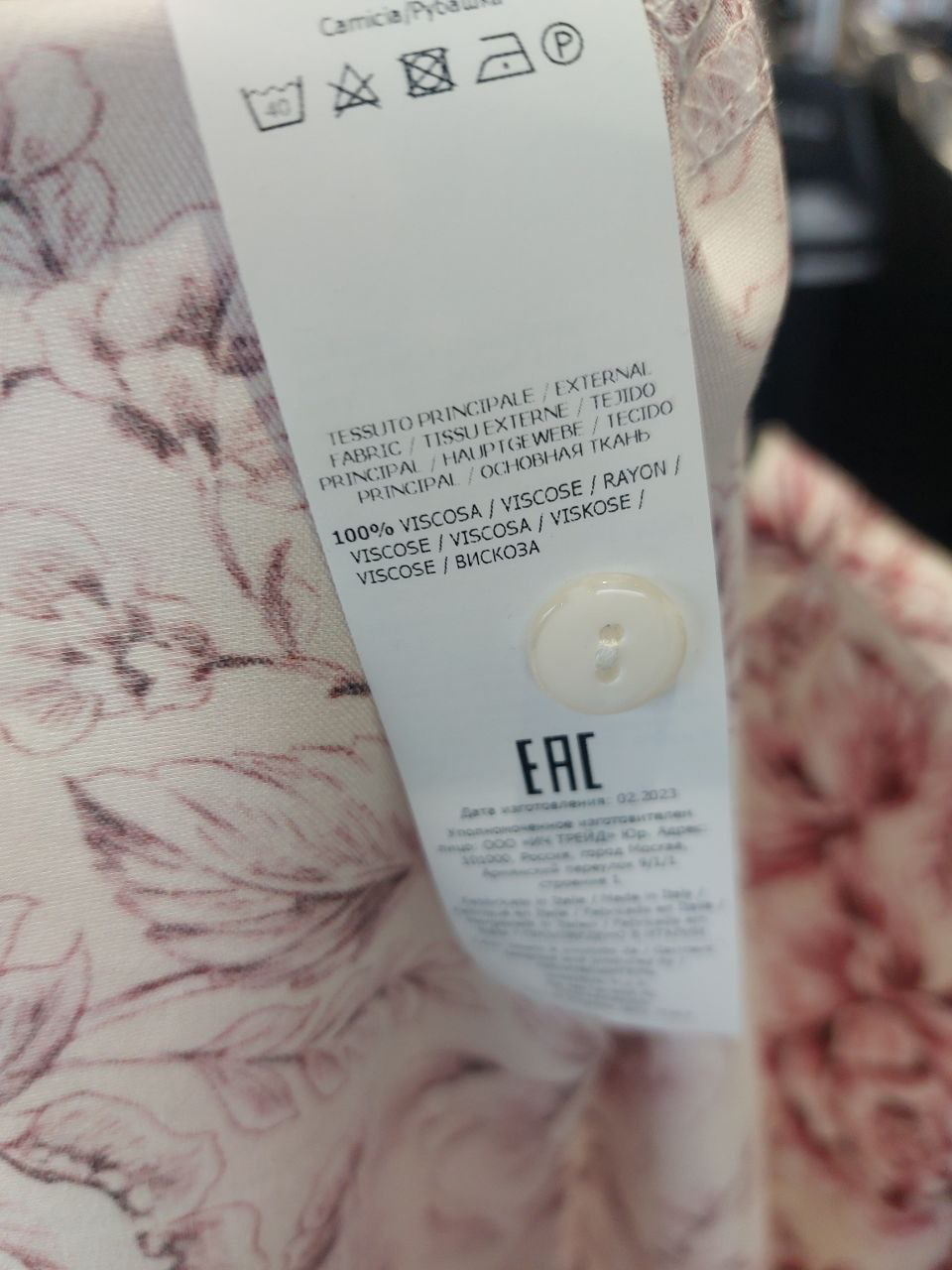This image captures a close-up of a large white tag attached to a garment, potentially made more prominent by the close view. The tag features a two-hole white button stitched onto it, affixing it to the fabric. The tag is printed in multiple languages, prominently displaying phrases like "100% viscosa," "viscose," and "rayon" to indicate the material composition. The English text visible includes "external fabric." The label further carries the bold letters "EAC," followed by several lines of black print that remain unreadable, possibly in a language resembling Russian.

The background shows part of a fabric with a cream-colored base adorned with dark red or pink floral and leaf patterns. This fabric might be upholstery or a piece of clothing, but its exact nature is unclear. Additionally, symbols on the tag provide care instructions, suggesting that the fabric should not be put in the dryer but can be ironed. The scene also includes a small, mostly black square in the upper right corner, adding a contrasting detail to the composition.